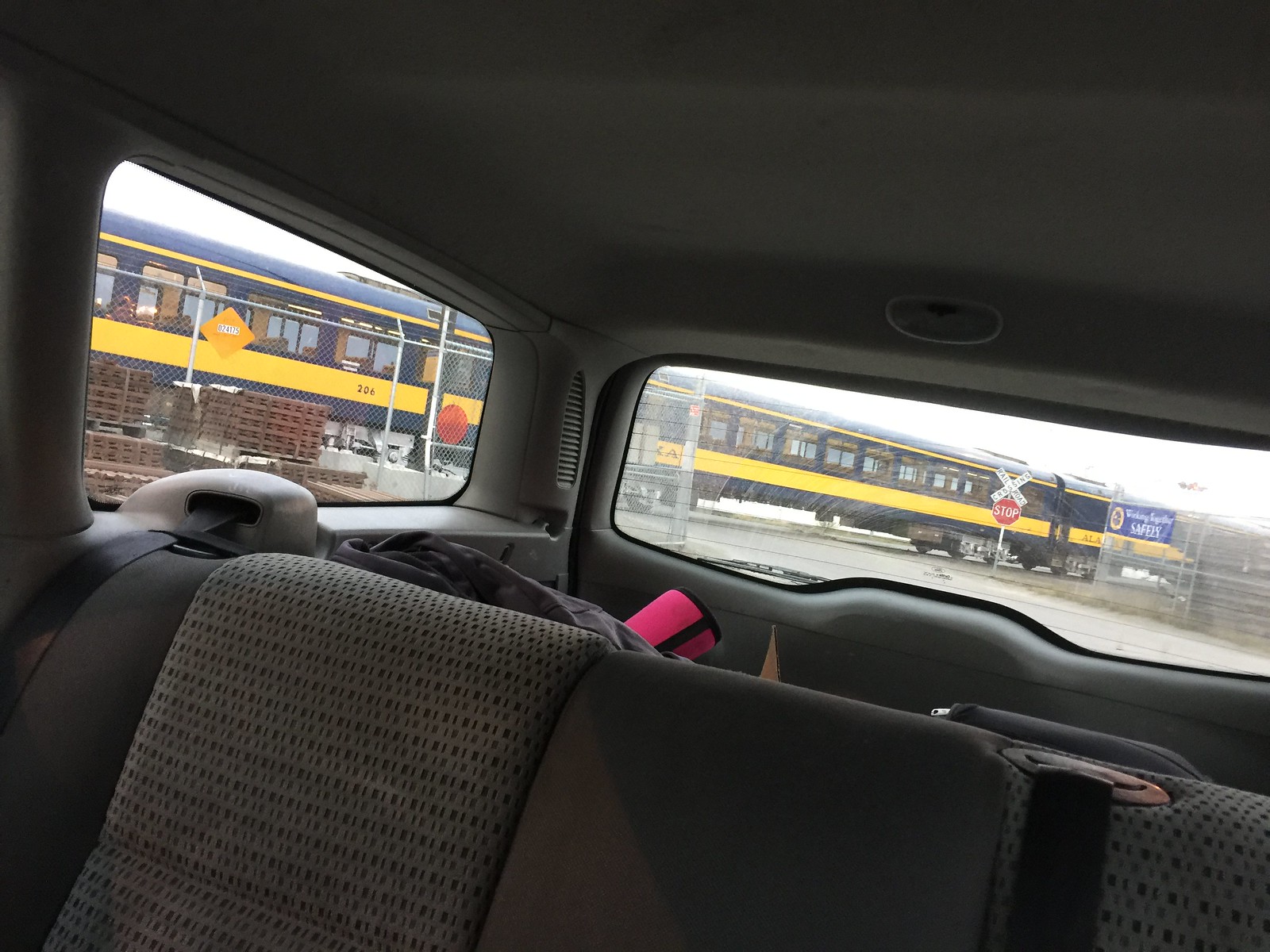The photograph captures the interior of a somewhat dirty vehicle with dark gray or black fabric bench seats displaying a faded pattern, where seat belts are visible. The image is taken from the front seat, looking towards the back seat and the cargo hold area. A notable pink koozie is peeking over the back seat, adding a splash of color. Through the back and rear passenger windows, one can see a blue and yellow passenger train with visible windows and a few passengers inside, although it's not crowded. The train appears to be either stationary or moving, as its direction is unclear. Also visible are a stop sign and a railroad crossing X sign, indicating the presence of a train crossing. Some items such as a yoga mat are barely visible within the trunk space, hinting at the presence of other baggage.